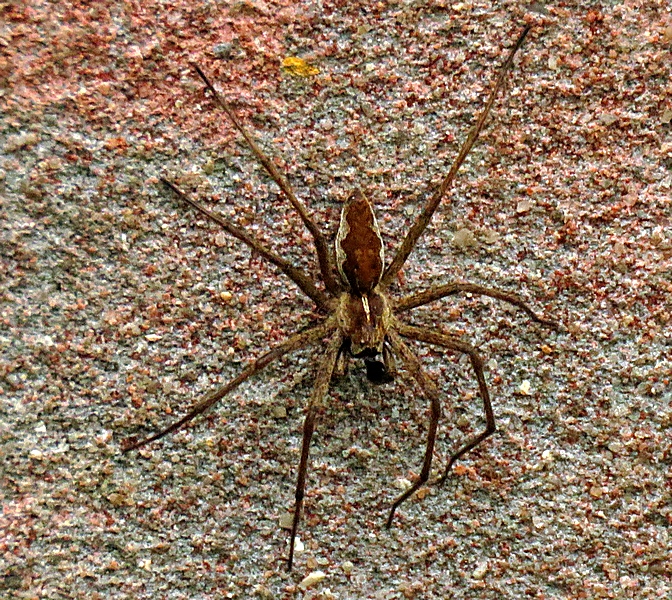This detailed photograph presents a slightly wide rectangular, aerial view of a spider positioned on what seems to be a rock or tree bark surface, flecked with green moss, red, brown, and yellow hues. The spider, centrally located and facing downwards, has a distinctively detailed body and legs. The body consists of two main parts: the larger, almond-shaped abdomen, which is dark brown with a golden-colored border, and a smaller, thicker thorax with a golden stripe running across. This complex pattern also includes whitish edges near the intersection of the thorax and abdomen, creating a visually striking contrast.

The creature's eight long, slender legs show varying degrees of extension and curvature. On the right side, one leg is fully stretched towards the top right corner, while the others are more curved. On the left side, all four legs are fully stretched and evenly spread apart. The legs' differing positioning accentuates the spider's menacing presence as it rests on the surface.

Despite the close-up view, only two or three of the spider's eyes are discernible, adding to the detailed realism of this photograph which captures the spider's natural habitat and intricate body structure, making it a compelling display of nature's intricacies.